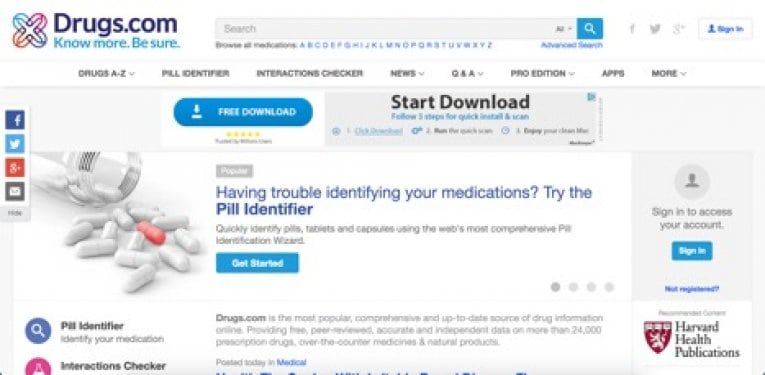This image is a screenshot from the website Drugs.com, which has a clean, white background. In the upper left corner, there's a distinctive, star-shaped symbol featuring a rainbow gradient with colors including teal, orange, purple, blue, pink, and red. Beside this symbol is the site's name, "Drugs.com," followed by the tagline, "No more be sure." In the upper center of the image, there's a search bar, while to its immediate right are social media icons for Facebook, Twitter, and Google. Further to the right in the upper corner, there is a "Sign In" button.

Beneath the Drugs.com logo, a navigation menu starts on the left with options such as "Drugs A to Z," followed by "Pill Identifier," "Interactions Checker," "News," "Q&A," "Pro Edition," "Apps," and "More." In the center of the page, there is a prominent "Free Download" button labeled "Start Download," suggesting content that might relate to a promotional offer or ad. Below this button is an article headline, "Having trouble identifying your medications? Try the pill identifier."